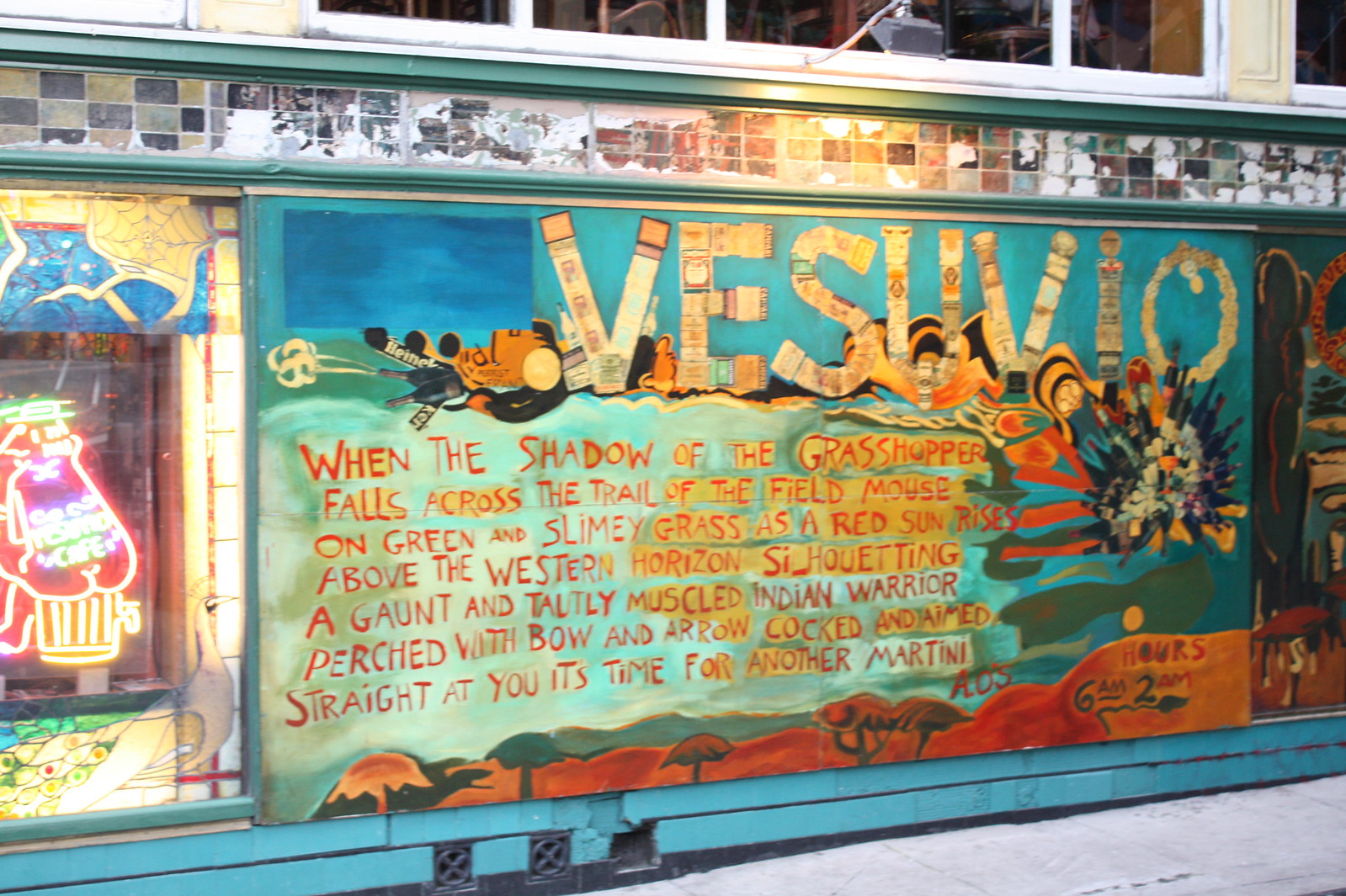The side of this building features a vibrant mural with various elements competing for attention. On the left, there's a white neon sign, which is somewhat difficult to decipher but could be depicting someone sitting on a trash can. The rest of the wall is adorned with colorful, abstract artwork, dominated by a multicolored sign and a detailed mural.

The background of the mural is a mix of blue and orange hues, creating a striking contrast with the gold and orangey lettering of the word "Vesuvio" painted prominently at the top. Below this, in orange letters set against a green background, a surreal and poetic inscription reads: "When the shadow of the grasshopper falls across the trail of the field mouse on green and slimy grass as a red sun rises above the western horizon, silhouetting a gaunt and tautly muscled Indian warrior perched with a bow and arrow cocked and aimed straight at you, it's time for another martini."

Further details of the mural include lemon and blue tiles at the top, abstract symbols at the bottom that resemble either jellyfish or umbrellas in orange, and dark letters on the bottom right corner stating the hours of operation: "Hours: 6 a.m. to 2 a.m." with "a.m." emphasized in red. This intricate mural transforms the side of the building into a vibrant, eclectic canvas blending text, imagery, and abstract art.